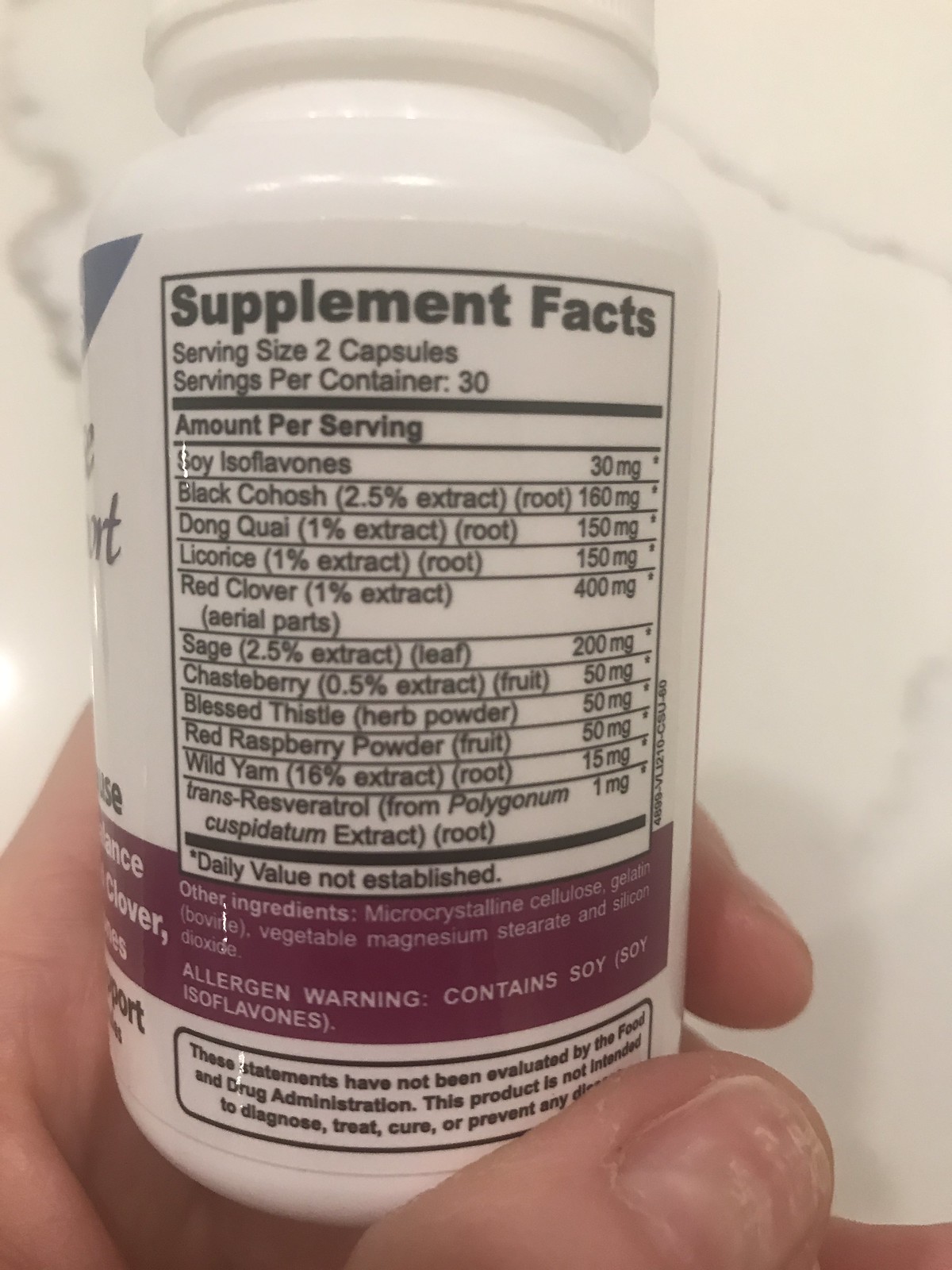A white bottle of vitamins or supplements featuring a detailed label that lists supplement facts. The label highlights a serving size of two capsules and indicates that the bottle contains 30 servings. Key ingredients include microcrystalline cellulose, gelatin, vegetable magnesium stearate, and silicon dioxide, with an allergen warning noting the presence of soy. The supplement comprises numerous herbal components such as Black Cohosh Root, Dong Quai, Licorice, Red Clover, Sage, Chasteberry, Blessed Thistle, Red Raspberry, Wild Yam, and Transresveratrol. Additionally, the daily values for these ingredients have not been established.